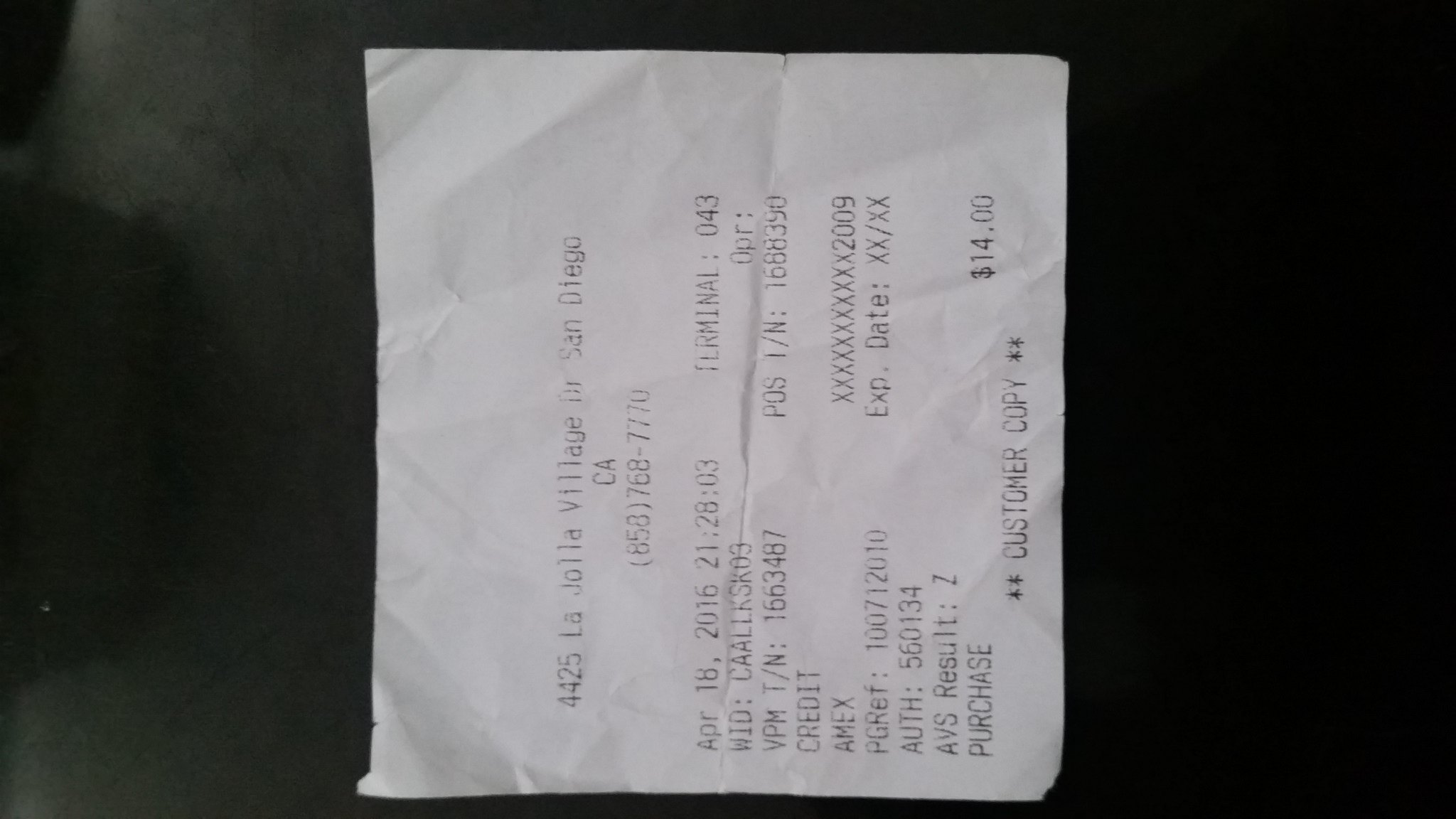In the image, there is a small, crinkled, white customer copy receipt placed horizontally on a completely black surface, rendering its information vertical. The receipt appears heavily crinkled, particularly in the middle, creating an impression of a rip that isn't actually there. The print on the receipt is black and slightly faint. The top of the receipt displays part of an address, mentioning "4425 La Jolla Village, San Diego, California". It also includes a phone number that is mostly obscured. The receipt shows a total purchase amount of $14, which was paid by credit card. The bottom of the receipt is oriented on the right, and the top is on the left, rotated 90 degrees from the upright position.